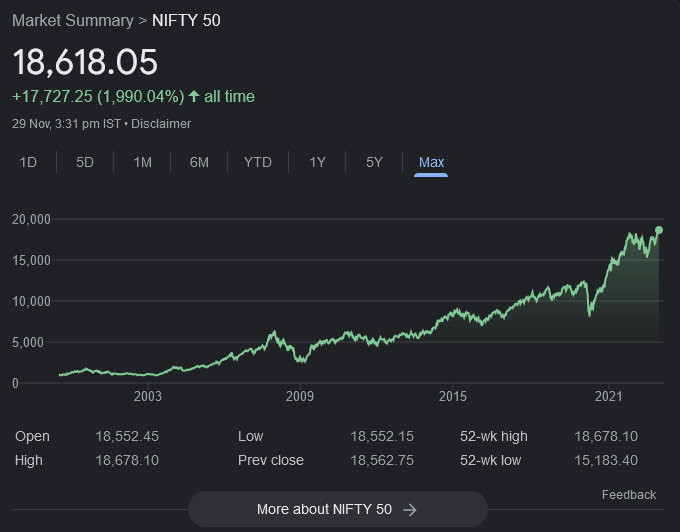The image displays a detailed graph of the NIFTY 50 stock index against a dark black background. At the top, the header "Market Summary" is shown in dark grey, followed by a greater than sign (>). In bold white text, the index name "NIFTY 50" is clearly labeled alongside the current value, "18,618.05". Below this, in bright green, it indicates a significant gain with "+17,727.25" and "$17,727.25" noted next to it. Additionally, the percentage increase of "1,990.04%" is also highlighted in green, accompanied by an upward arrow symbol, signaling an all-time high.

Beneath this, in grey text, the date and time are provided: "29 NOV" (November 29) and "3:31 PM IST", followed by a grey arrow pointing towards a disclaimer. 

There are multiple tab options for viewing the graph: 
- "1D" (one day)
- "5D" (five days)
- "1M" (one month)
- "6M" (six months)
- "YTD" (year to date, all capitalized)
- "1Y" (one year)
- "5Y" (five years)
- Finally, "MAX", displayed in cyan blue with a cyan blue line beneath it to indicate selection.

The left side of the graph shows a vertical scale ranging from 0 to 20,000 in 5,000 point increments. The graph itself is depicted in dark green, starting below 5,000 and rising to just shy of 20,000. Along the bottom of the graph, key years are marked: 2003, 2009 (showing fluctuations), 2015 (a general upward trend), and 2021 (a brief downward trend before resuming an upward trajectory).

On the lower left, specific stock details are shown:
- Open: $18,552.45
- Low: $18,552.15
- 52 Week High: $18,678.10
- High: $18,678.10
- Previous Close: $18,562.75
- 52 Week Low: $15,183.40

Additionally, there is an oval with bold white text stating "More about NIFTY 50", accompanied by a grey arrow pointing to the right. Just beyond this is a "Feedback" option, also on the right.